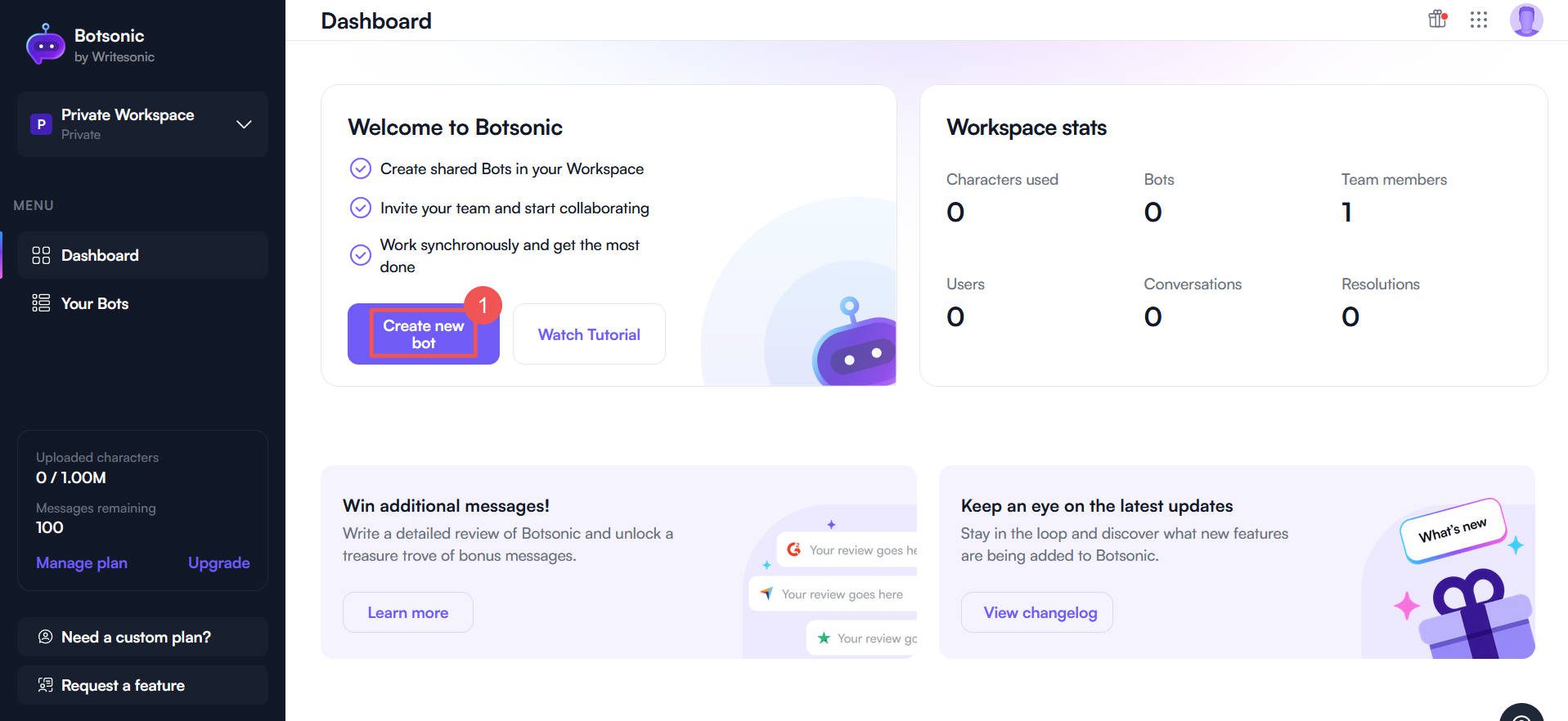**Screenshot of the BotSonic Website**

The image displays a screenshot from a website with a clean, white background complemented by elements of pale lilac. On the left side, there is a black navigation bar featuring a small purple alien-like character with two white dots for eyes at the top corner. The text "BotSonic" appears next to this character. Below it, there is a purple square containing a play button and the label "Private Workspace." This section has a dropdown option indicated by a small "P".

Further down the navigation bar, the word "Menu" is displayed, followed by the items "Dashboard" and "Your Bots". Below these items, there is some text in pale grey, which is difficult to read, indicating "0 out of 1 million." There is another grey item below this that reads "100." Further down, there is a purple button labeled "Manage Plan" and, to its right, a button labeled "Upgrade." Centered at the bottom of the column is the text "Need a Custom Plan or Request a Feature."

On the right side, the main section of the site is visible. In the top left corner, the word "Dashboard" is displayed. Towards the right, you have the "Home" button, a "Menu" option, and a profile picture. The main area features four prominently outlined rectangular blocks arranged in a grid format. 

The first block, titled "Welcome to BotSonic," includes three points listed below it and a purple button labeled "Create New Bot." Next to it, on the right, is another block titled "Workspace Stats," indicating information about "Team Members." Below these, the third block on the left is labeled "Win Additional Messages" and includes a "Learn More" option. To its right, the fourth block is titled "Keep an Eye on the Latest Updates," with a gift icon popping up from the bottom right corner. The "Welcome to BotSonic" block also features a white button labeled "Watch Tutorial," and the little bot icon peeks out from the bottom right corner of this section.